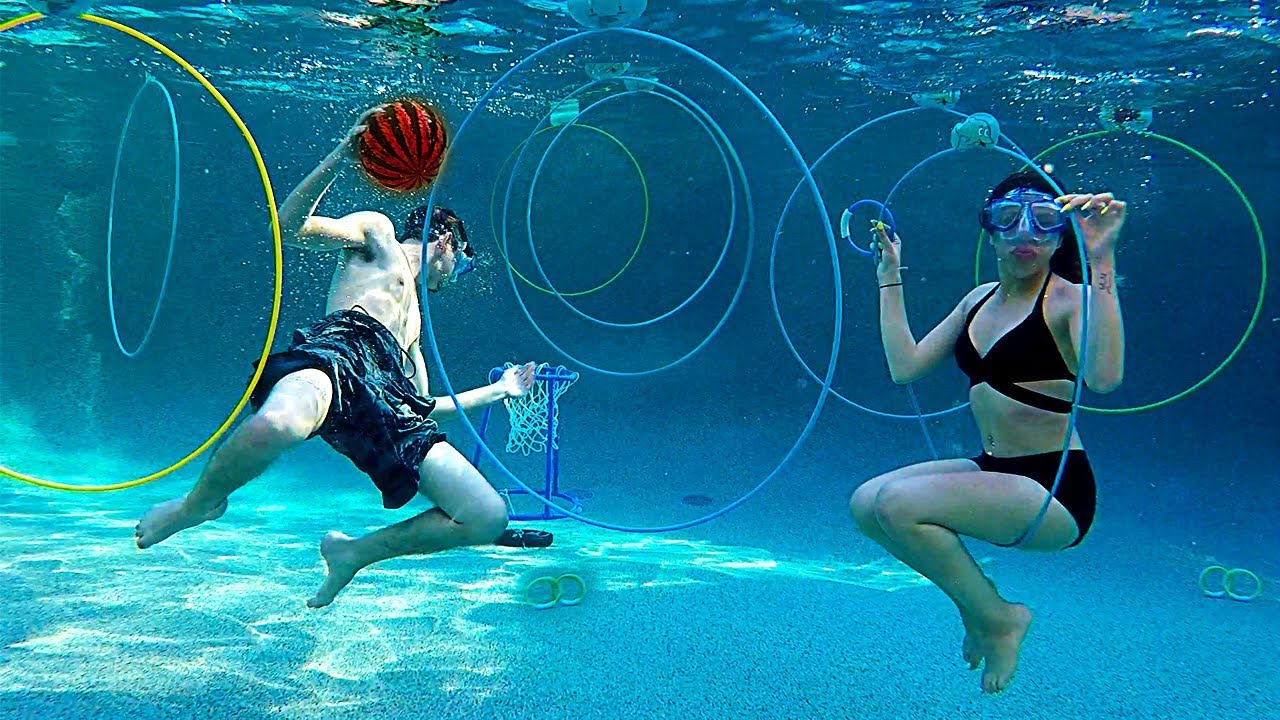In this vivid underwater photograph, two individuals are immersed in a playful, aquatic scene within a pool that might be part of an aquarium, as suggested by the glass wall enclosing the space. The backdrop is a mesmerizing, crystal blue water illuminated by the light penetrating from above. 

On the right, a woman is captured seated inside a blue and green hoop, which rests beneath her legs. She is identifiable by her black two-piece bathing suit, diving mask, and accessories, including a tattoo and bracelet. Around her, numerous colorful hoops—white, orange, blue, and yellow—are suspended in the water, creating a vibrant, dynamic environment.

To her left, a young man, dressed in blue swim trunks and also sporting a diving mask, prepares to slam dunk a distinctive red and black basketball into a hoop anchored to the bottom of the pool. A variety of hoops, some settled on the pool floor, add to the playful ambiance.

Both individuals appear to be holding their breath, engrossed in their activities, contributing to a truly engaging, underwater spectacle of sports and playfulness.